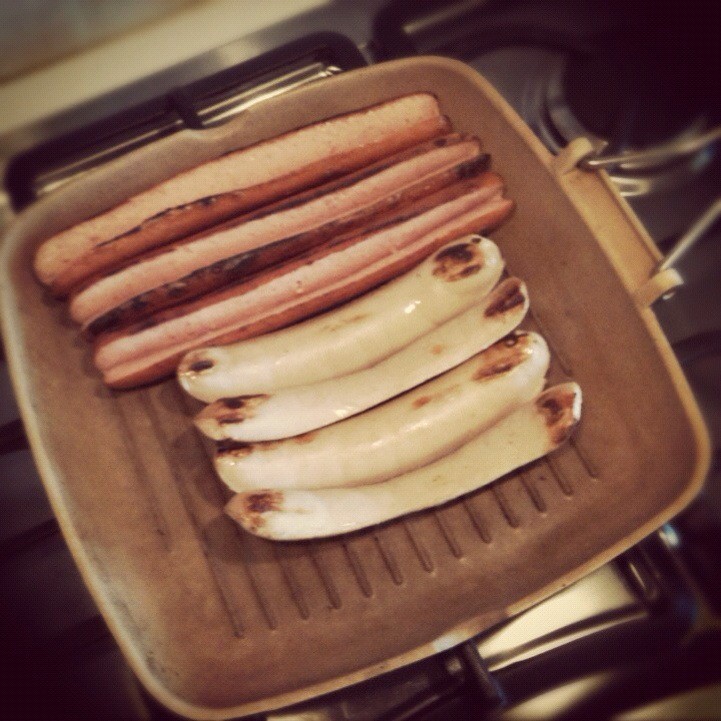This is a square Instagram-style photograph featuring a grey, ridged skillet with a metal, foldable handle, likely intended for camping. The image has a sepia-toned filter that produces a blurry effect around the edges, emphasizing the center more clearly. The skillet sits atop a gas burner from which some black grilling grates are visible.

Inside the skillet, three long hot dogs, split lengthwise to create a V-shaped opening, take up most of the space. These hot dogs have distinct char and grill marks, giving them a pinkish-brown hue. Additionally, four smaller, whitish sausages, also marked with grill lines but maintaining their shape without melting, are arranged around the larger hot dogs. The setting is otherwise plain, with chrome elements visible in the background.